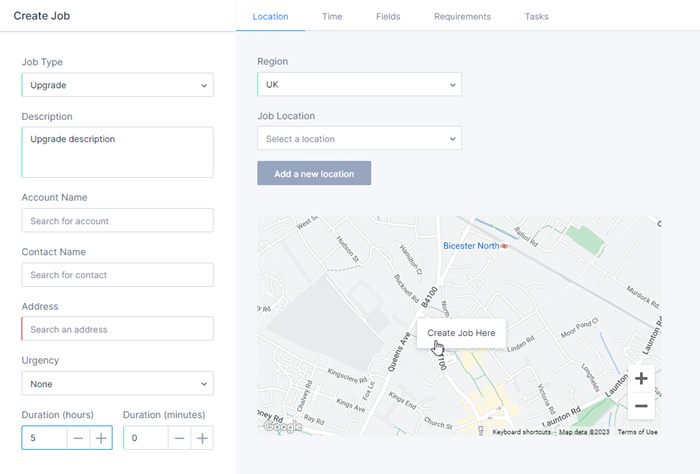The image depicts a job creation interface within an application or platform. The screen is divided into two primary sections: a gray section on the right and a white section on the left. 

### Top Section:
- **Top Left**: The words "Create Job" appear in black.
- **Top Right**: Contains headings labeled "Location," "Time," "Fields," "Requirements," and "Tasks," with "Location" underlined in blue.

### Right Section (Gray Background):
- **Region**: Displayed with a dropdown box currently set to "UK."
- **Job Location**: Includes a dropdown box labeled "Select a location," and a button labeled "Add a new location" in white text on a gray background.
- **Map**: A map is centered, showing various place names including "Bicester North," "Queens Avenue," "B4100," "Hamilton Court," "Hudson Street," "Kingsclare Road," "Kings Avenue," "Victoria Road," and "Lawnton Road." In the center of this map, a white button labeled "Create a job here" is being hovered over by a white hand icon (mouse cursor).

### Left Section (White Background):
- **Job Type**: Display area labeled "Upgrade."
- **Description**: Area for job details.
- **Account Name**: Field to "Search for accounts."
- **Contact Name**: Field to "Search for contact."
- **Address**: Field to "Search an address."
- **Urgency**: Set to "None."
- **Duration**:
  - **Hours**: Indicated as "5."
  - **Minutes**: Indicated as "0."

This detailed breakdown captures all the visual elements and text present in the image.